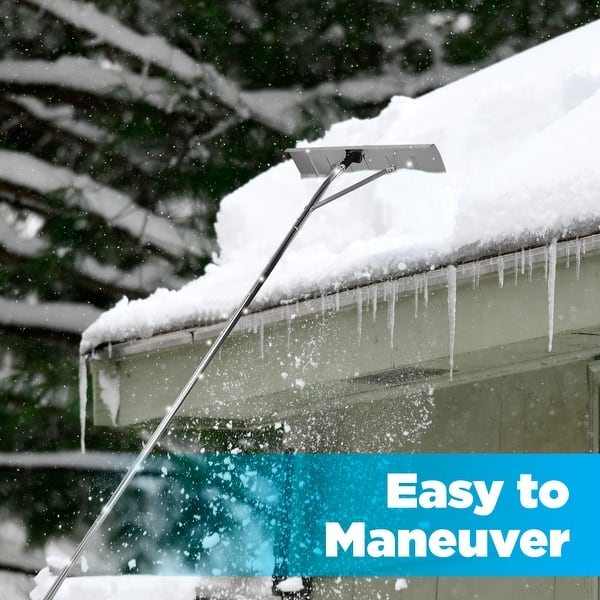The photograph captures a snowy outdoor scene during daytime, focusing on the corner of a house roof blanketed in thick white snow. Icicles dangle from the eaves, evoking the chilly atmosphere. Emerging from the lower left corner of the image is a long, silver steel rod, gleaming with a sleek, metallic finish. This tool boasts a flat, rectangular blade at its top, designed to efficiently scrape snow off the roof. Snowflakes appear to be falling delicately, adding to the wintry ambiance. In the background, snow-covered pine trees and branches are visible, enhancing the serene, snowy landscape. The bottom right corner of the photo features a gradient blue banner with bold white text that reads "Easy to Maneuver," hinting at the tool's user-friendly design.